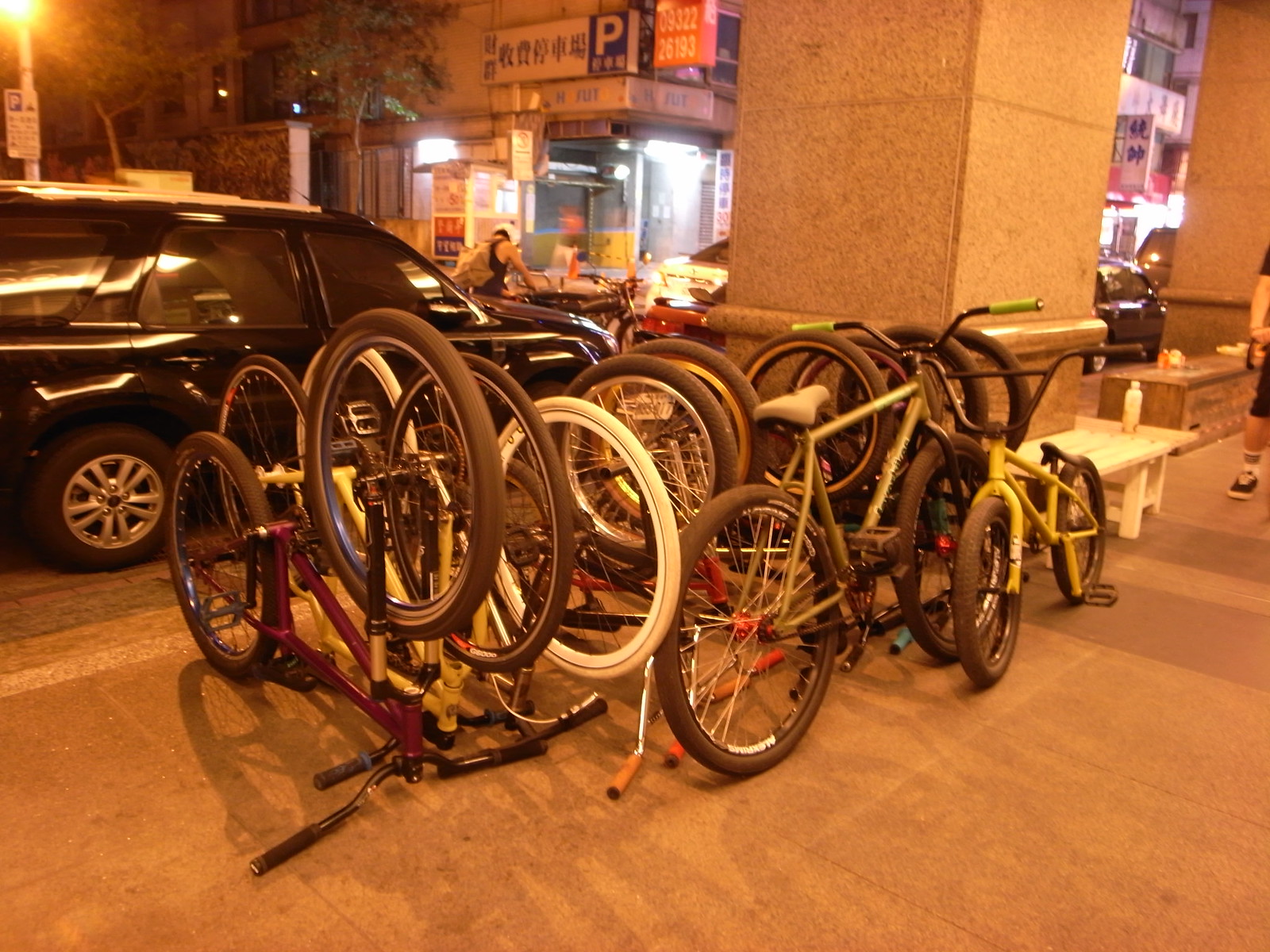In this color photograph with an orange tint, likely caused by a streetlight illuminating the scene at night, a bunch of bicycles are bunched up together on a sidewalk, just off the side of the road. The bicycles, ranging in colors and styles, are arranged almost in a pile, some intentionally upside down with their handlebars pointing towards the concrete. Specifically, there are three prominent upside-down bikes: a pink one, a yellow one, and a black one, with several others blocking the view of additional upside-down bikes. An upright green bike with a white seat and a small yellow child's bike are also visible among the pile.

In the foreground to the right, there's a pedestrian's right arm and right leg, dressed in a black shirt and black shorts, extending into the frame. Directly to the left of this figure, a white bench with a water bottle on it can be seen, along with a brown bench farther back, which has some items placed on it. A large concrete pillar stands behind the white bench.

The background reveals a busy commuter street in what appears to be a foreign city, given the signs with non-English characters above the storefronts and shops. A black SUV is driving up the street, in front of which a man sits outside a diner with its windows and possible shop lights visible. Additionally, there is a man riding a delivery bike, equipped with a backpack and a white helmet, blending into the lively street scene where several people can be seen walking by.